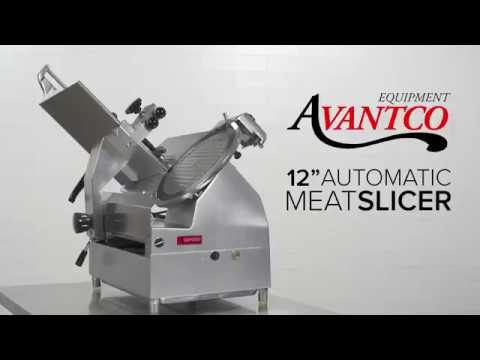This image serves as an advertisement for a 12-inch automatic meat slicer from Avantco Equipment. The rectangular image features black borders on the top and bottom, resembling widescreen television bars. On the right-hand side, the text "Equipment Avantco" is prominently displayed, with the 'A' stylized with a long curve extending from its bottom right. The word "Avantco" is written in red, while below it, in black letters, the description "12-inch automatic meat slicer" is provided. Dominating the left side of the image is the metallic meat slicer itself, perched on a matching metallic table. The slicer is silver-gray with black knobs, a power switch, and four short legs. It features a tray set diagonally and a circular saw-like blade intended for slicing meat, with adjustable settings for thickness and portion size. The entire scene is set against a clean white background, highlighting the sleek design of the slicer.